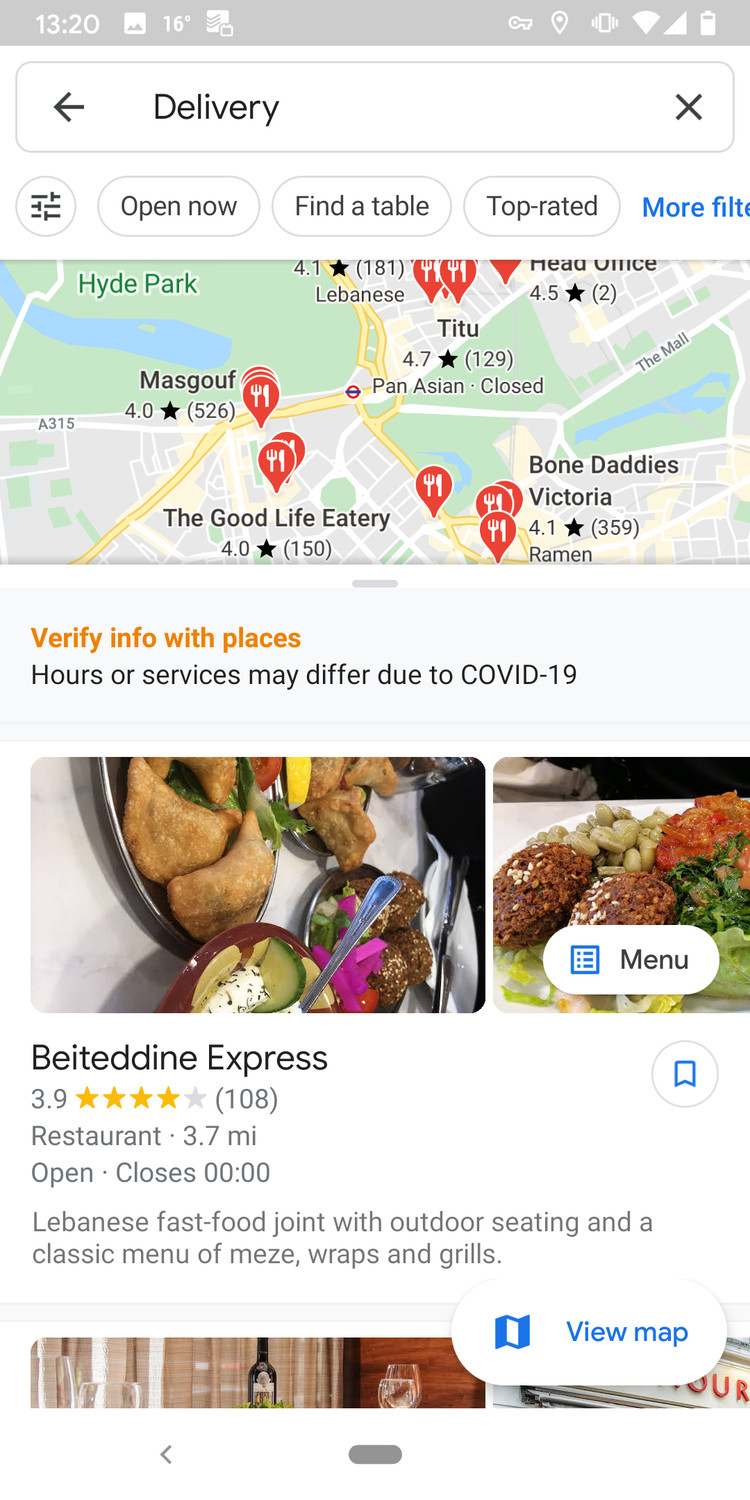The image displays a screenshot of a mobile device's interface. At the top left corner, the device's time reads 1:20 PM, and the weather app indicates a temperature of 16 degrees. The status bar is populated with various icons: a gallery icon, a VPN active icon, a location active icon, a vibration active icon, a Wi-Fi active icon, a fully filled network signal bar, and a battery status icon on the top right corner. The screen shows a search field exhibiting the word "delivery." Additionally, there is a map with marked locations, including MarsGov, The Good Life E3, and Bone Dirties.